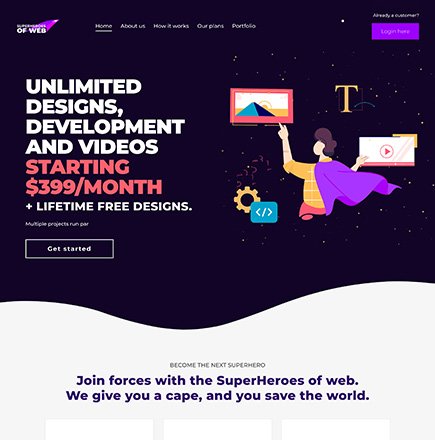The image is a screenshot of a website with a predominantly black background, transitioning to light gray at the bottom. A subtle curve runs through the center of the black portion. At the very top, partially obscured text is visible, including the legible phrase "of web." Purple lines emanate downwards from the top section. Below this, a navigation menu includes the options: Home, About Us, How It Works, Our Plans, and Portfolio. Additionally, there's a phrase "already us" that trails into illegibility, followed by a visible "log in here" prompt.

Prominently displayed in large white text in the central area is the phrase "UNLIMITED DESIGNS, DEVELOPMENT, AND VIDEOS." Directly below, in bold red capital letters, it states "STARTING AT $399 PER MONTH." This is followed by smaller but still capitalized text in white, "PLUS LIFETIME FREE DESIGNS." A clickable "Get Started" button is positioned beneath this text.

On the right side of the image, there’s a cartoon figure donning a purple cape, pointing towards various screens. The light gray bottom segment contains the motivational message, "Become the next superhero. Join forces with the SuperHeroes of Web," with "SuperHeroes" stylized with capital S and H. Encapsulating the theme, it concludes with, "We give you a cape, and you save the world."